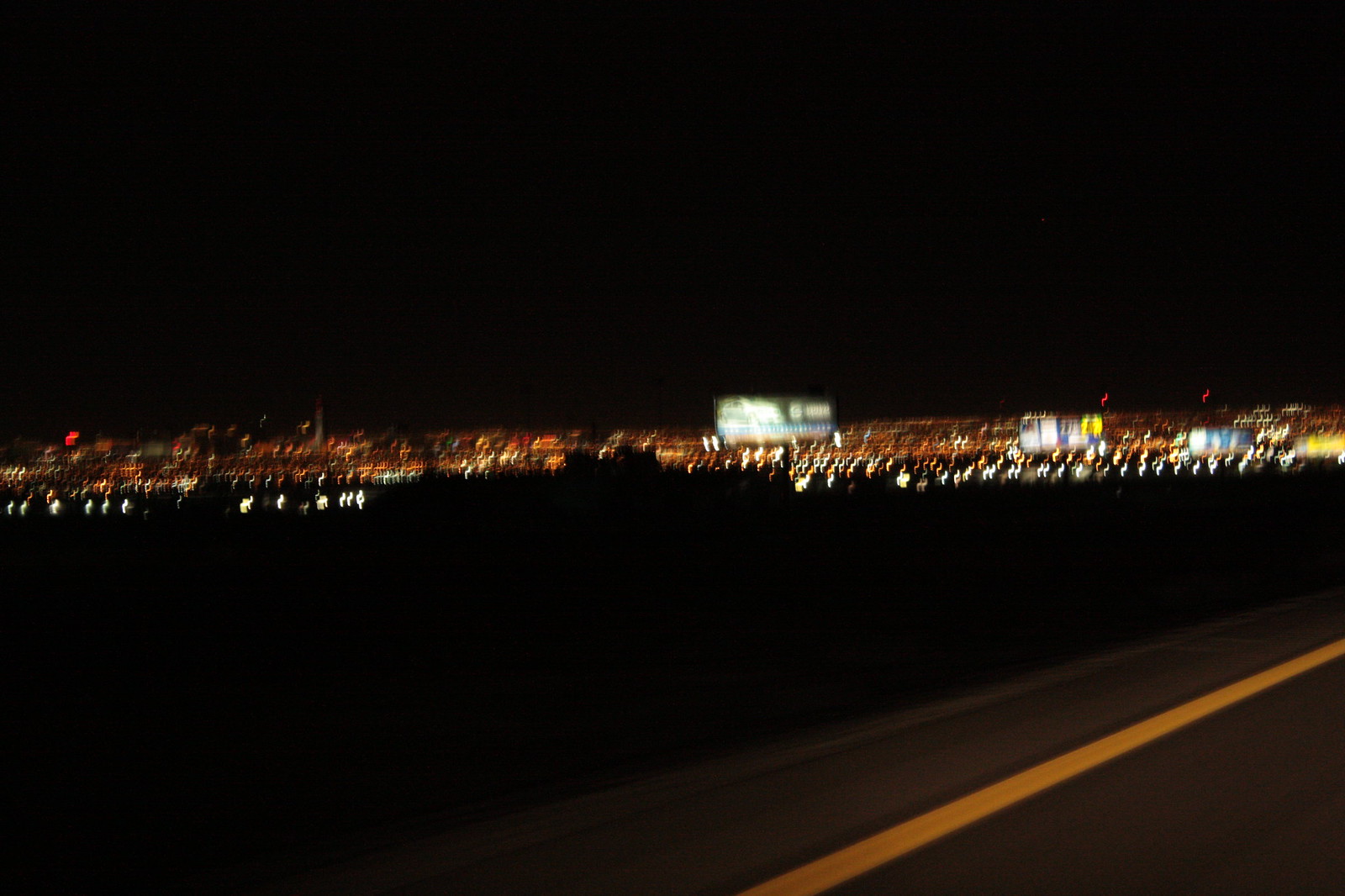This is a photograph of the Las Vegas skyline taken at night from a moving vehicle on the road. The image is blurry, emphasizing the motion. In the bottom right-hand corner, there is a yellow line indicating the shoulder of the road. The skyline features notable casinos like the Stratosphere and the Rio on the left, with a total of four visible billboards scattered near the highway. The illuminated cityscape spans the entire horizon, presenting a mix of bright and dimmer orange lights from buildings, neighborhoods, and streets in the background. The sky and the ground between the road and the city remain completely dark, highlighting the vibrant yet distant lights of the iconic Las Vegas skyline.